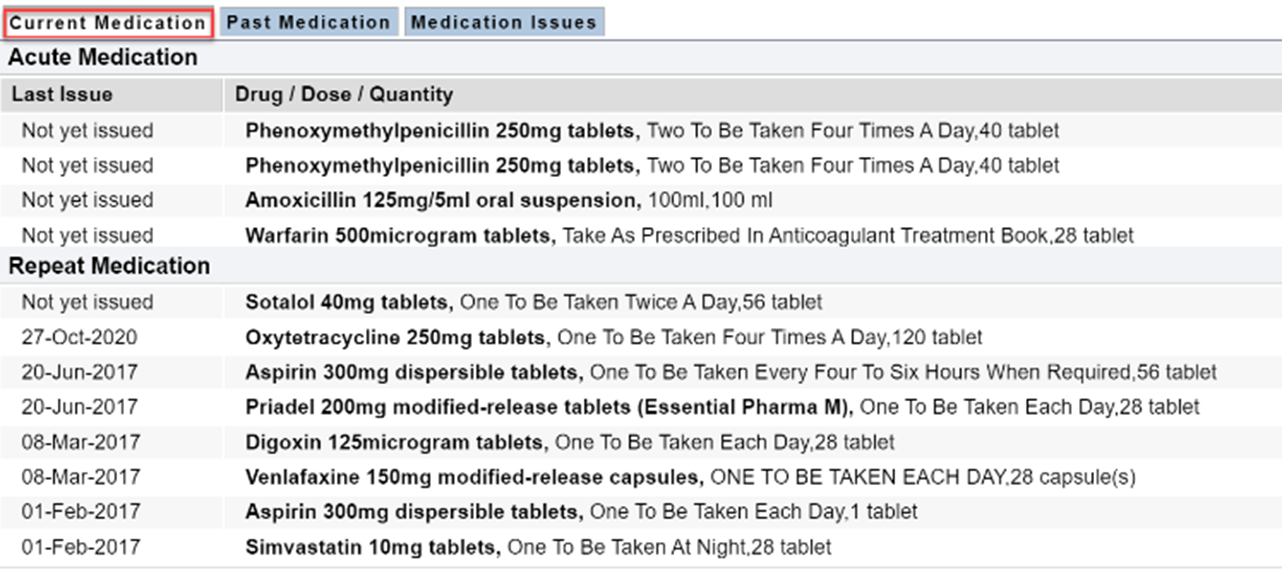"Screenshot of a Medication Management Website: The interface features three prominent banners labeled 'Current Medication,' 'Past Medication,' and 'Medication Issues.' The 'Current Medication' section is highlighted in a red box, while the others have a blue background. Within the 'Current Medication' section, it's categorized under 'Acute Medication,' listing the details as follows:

- **Last Issue**: Each medication has not yet been issued.
- **Medications**: 
  - *Phenoxymethylpenicillin*: Two entries of 250 mg tablets, with a dosage of two tablets to be taken four times a day, totaling 40 tablets.
  - *Amoxicillin*: One entry of 125 mg/5 mL oral suspension, with a volume of 100 mL.
  - *Warfarin*: One entry of 500 microgram tablets, with instructions to take as prescribed, listed as an anticoagulant treatment, and totaling 28 tablets.

At the bottom, there's a section for 'Repeat Medication not yet issued,' which includes eight listed medications with corresponding dates, years, and months."